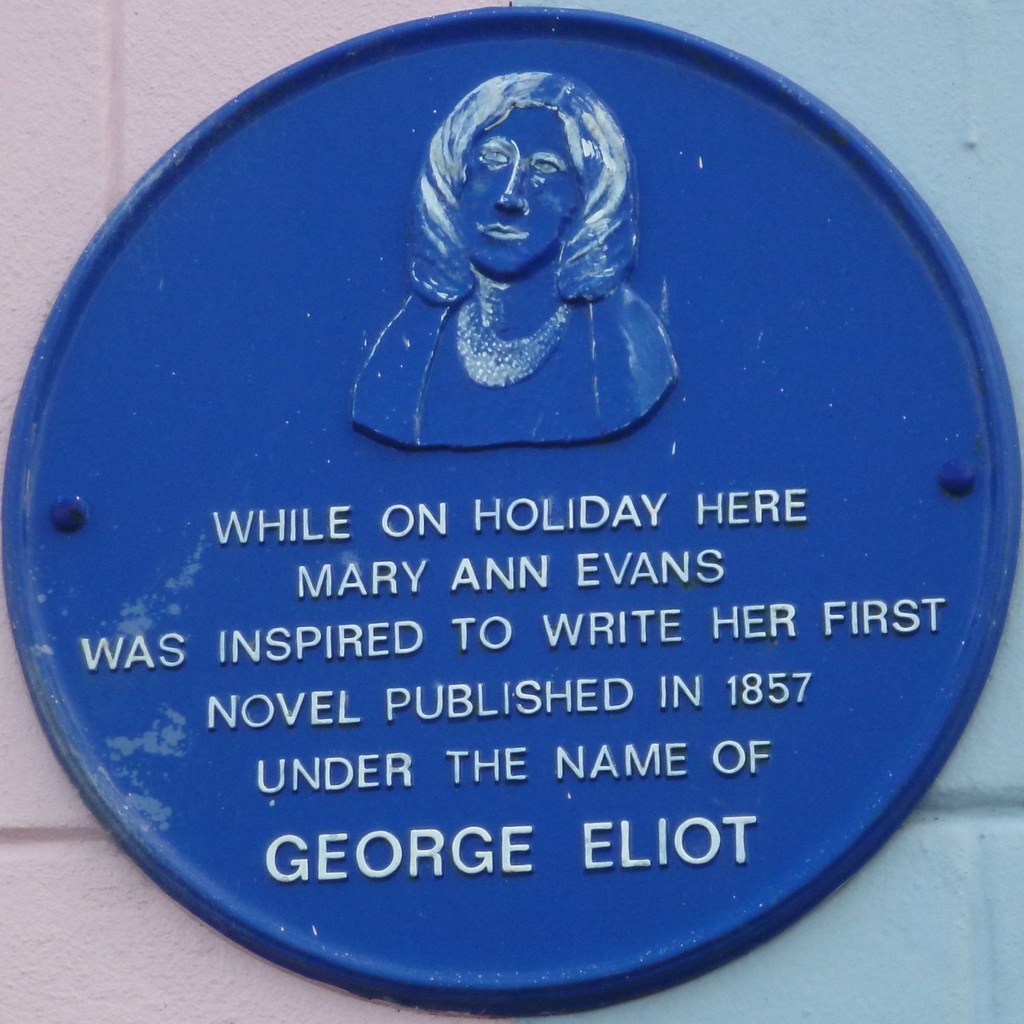Attached to a white-painted stone wall, there is a round, blue plaque securely fastened with bolts on either side. The plaque features raised, white-painted text that reads: "While on holiday here, Mary Ann Evans was inspired to write her first novel published in 1857 under the name George Eliot." Above the text, there is a carved portrait of a woman with shoulder-length hair, adorned with a thick necklace and wearing a simple top. The woman, presumably Mary Ann Evans, gazes slightly upward. The plaque stands out against the white building as daylight dims.